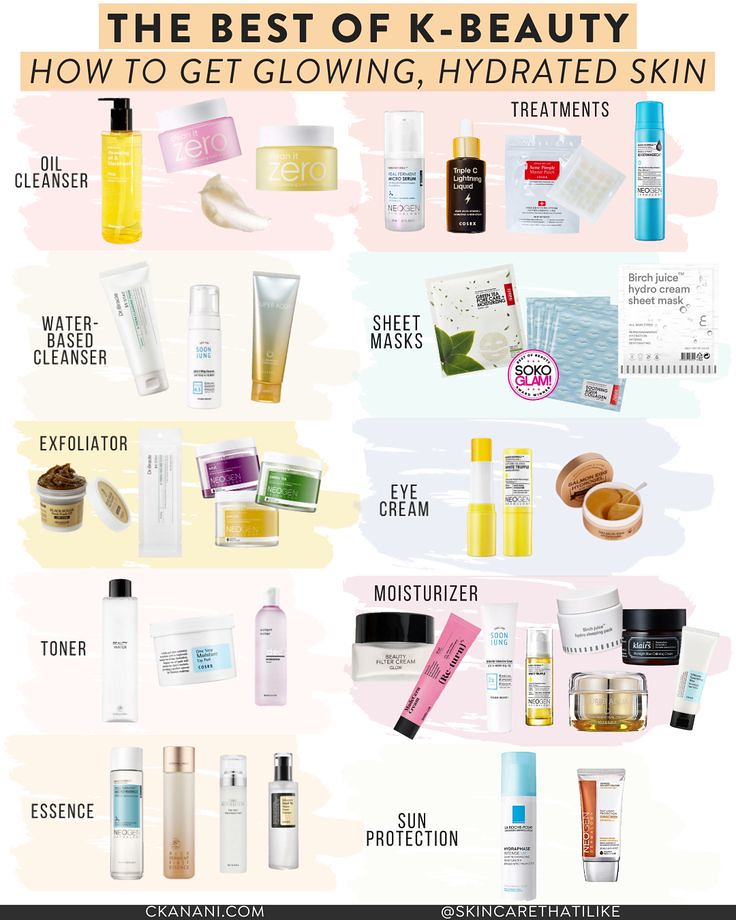**Detailed Caption for the Image:**

The color image showcases a comprehensive collection of popular K-beauty products, highlighting various steps to achieve glowing, hydrated skin. At the top, the text reads, "The Best of K-Beauty: How to Get Glowing, Hydrated Skin," introducing the diverse array of items featured.

1. **Cleansing Oils:**
   - A yellow bottle with a black pump.
   - A round pink container with a white lid labeled "Zero."
   - A golden container with a white lid, also labeled "Zero."
   - A smear of white substance beneath the mentioned containers.

2. **Treatments:**
   - A small, shiny white package with a square material on top.
   - A white bottle.
   - A black bottle with a gold cap labeled "Triple C Lightning Liquid."
   - A tall, blue bottle.

3. **Water-Based Cleansers:**
   - A white tube.
   - A white bottle.
   - A shiny gold and silver tube (text is unclear).

4. **Sheet Masks:**
   - A white packet with green leaves imagery.
   - Five blue packets with white kiss marks labeled "Soothing Aqua Collagen."
   - A white packet labeled "Birch Juice Hydro Cream Sheet Mask."
   - A "Best of Beauty SOKO Glam" circle between the left and middle masks.

5. **Exfoliators:**
   - An open jar with a brown substance.
   - A white square bottle.
   - Three small glass jars with white lids: one with a purple label, one with a green label, and one with a yellow label (text is too small to read).

6. **Eye Cream:**
   - A rolled-up yellow tube with a white middle, showing a golden substance inside, partly labeled "NEOGEN."
   - A small round container with a brown lid placed behind it, containing a brown substance and a small plastic spoon/spatula.

7. **Toners:**
   - A tall white bottle with a black cap.
   - A round container with a white lid and a blue and white label.
   - A lavender bottle with a white cap (text is too small to read).

8. **Moisturizers:**
   - A white jar with a black lid labeled "Beauty Filter Cream."
   - A pink tube with a black cap labeled "Re-turn."
   - A white tube labeled "Soon Sung."
   - A small golden-colored glass bottle.
   - A round white container and a round black container.
   - Two small glass containers with a gold substance inside.
   - A white tube with a blue label (text is too small to read).

9. **Essences:**
   - A tall clear bottle.
   - A tall brown bottle.
   - A tall white bottle.
   - Another tall clear bottle (text is too small to read).

10. **Sun Protection:**
    - A white bottle with a blue cap labeled "LA ROCHE-POSAY."
    - A brown and white tube with a silver cap.

At the bottom, the image is labeled "CKANANI.com at Skincare That I Like," indicating the source.